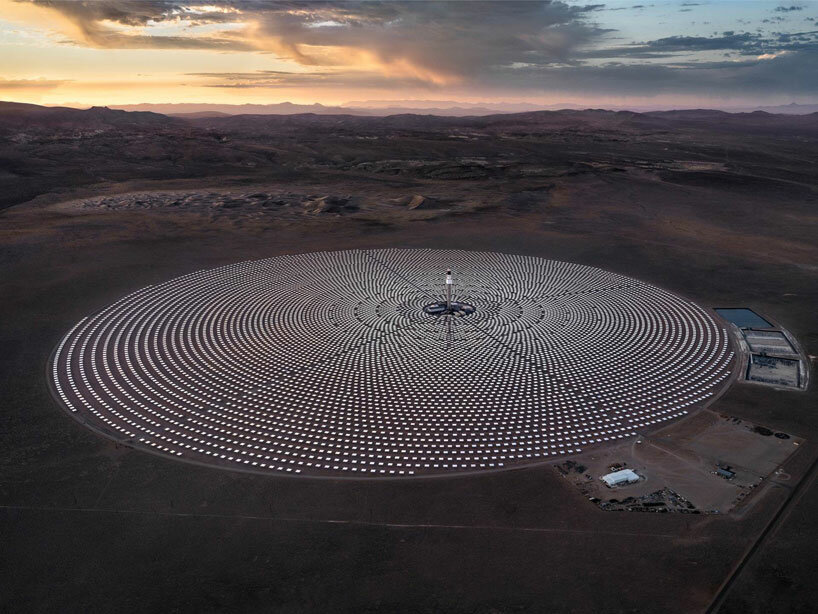The photograph captures an aerial view of a vast, circular science structure situated in a desolate desert landscape. The central feature of the image is a large circular depression filled with rows of small, silver dots extending from the center to the edges, creating a striking visual pattern. At the very center of this circle is a silver pole with a white top, from which three wires extend outward. 

Surrounding the structure, the arid ground is packed hard and barren, characterized by red sand and rocks. To the right of the circular formation, three prominent squares can be seen; the topmost contains blue water, while the other two are empty, accompanied by a small parking lot and building complex nearby. 

In the background, the terrain gradually rises into distant mountains capped by an expansive sky. The sky features a mesmerizing gradient from a yellow and orange sunset on the left, transitioning to a reddish-pink hue and finally a deep blue on the right. Thick clouds with shades of gray, white, and reflections of pink and yellow are scattered across the sky, adding depth and drama to the scene. The overall color palette of the image is somewhat muted, contributing to a slightly eerie, abandoned atmosphere.